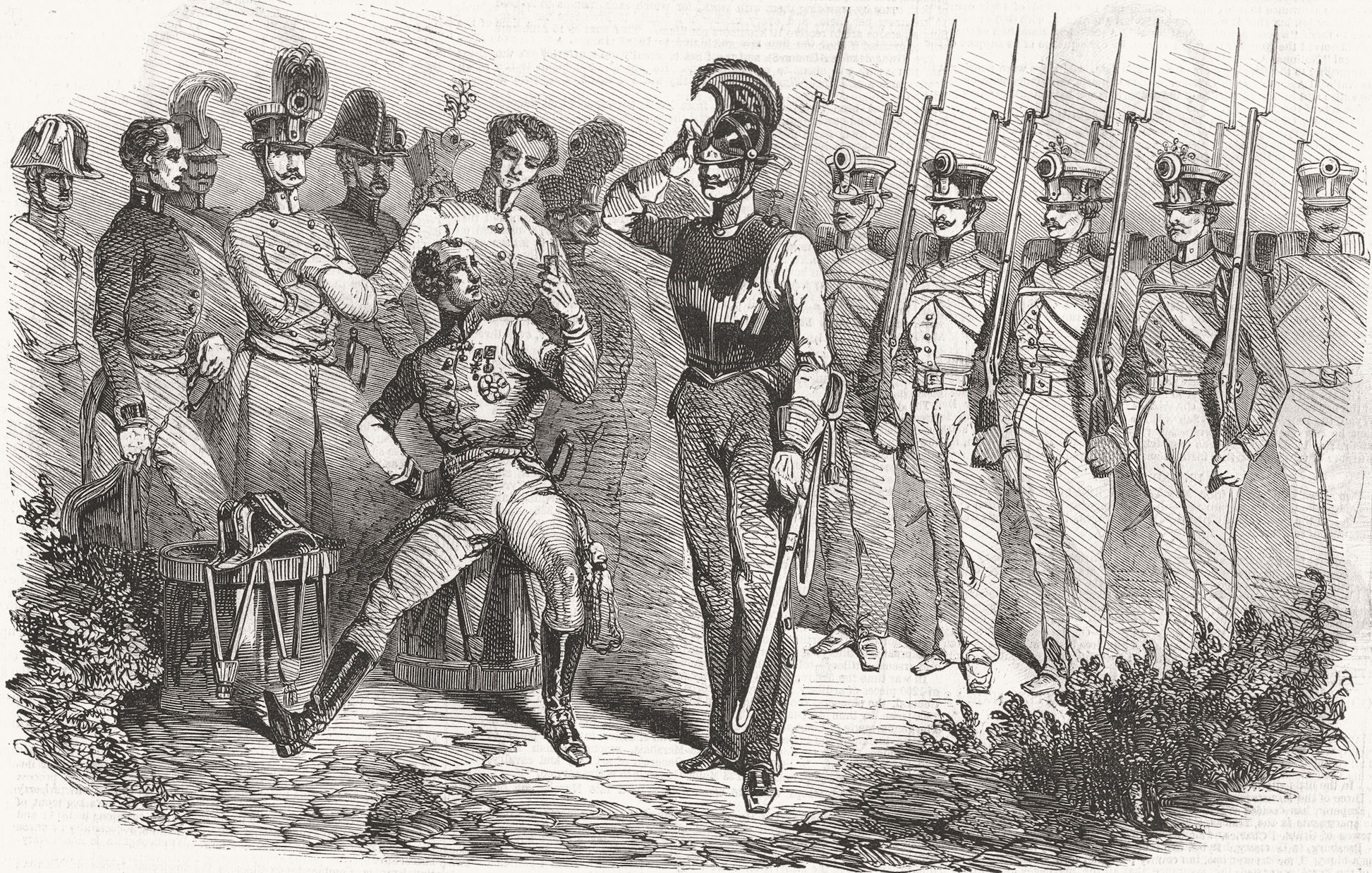This black and white line ink illustration, likely from the early 1800s, depicts a detailed military scene in an open area. On the right, a rank of five soldiers stands at attention with their leader in front, saluting. Each soldier is equipped with a rifle that has a spike bayonet attached. The leader, distinguished by a helmet and metal breastplate, also carries a sword saber at his side. On the left side of the image, a group of noblemen or officers, dressed in posh buttoned-up jackets, tight slacks, and black boots, engage in conversation. One man, seated on a drum with another drum beside him, looks up while possibly holding a cup or gesturing toward the military leader. The scene is enriched by the officers' elaborate hats and plumes, emphasizing the formal and ornate nature of their attire.